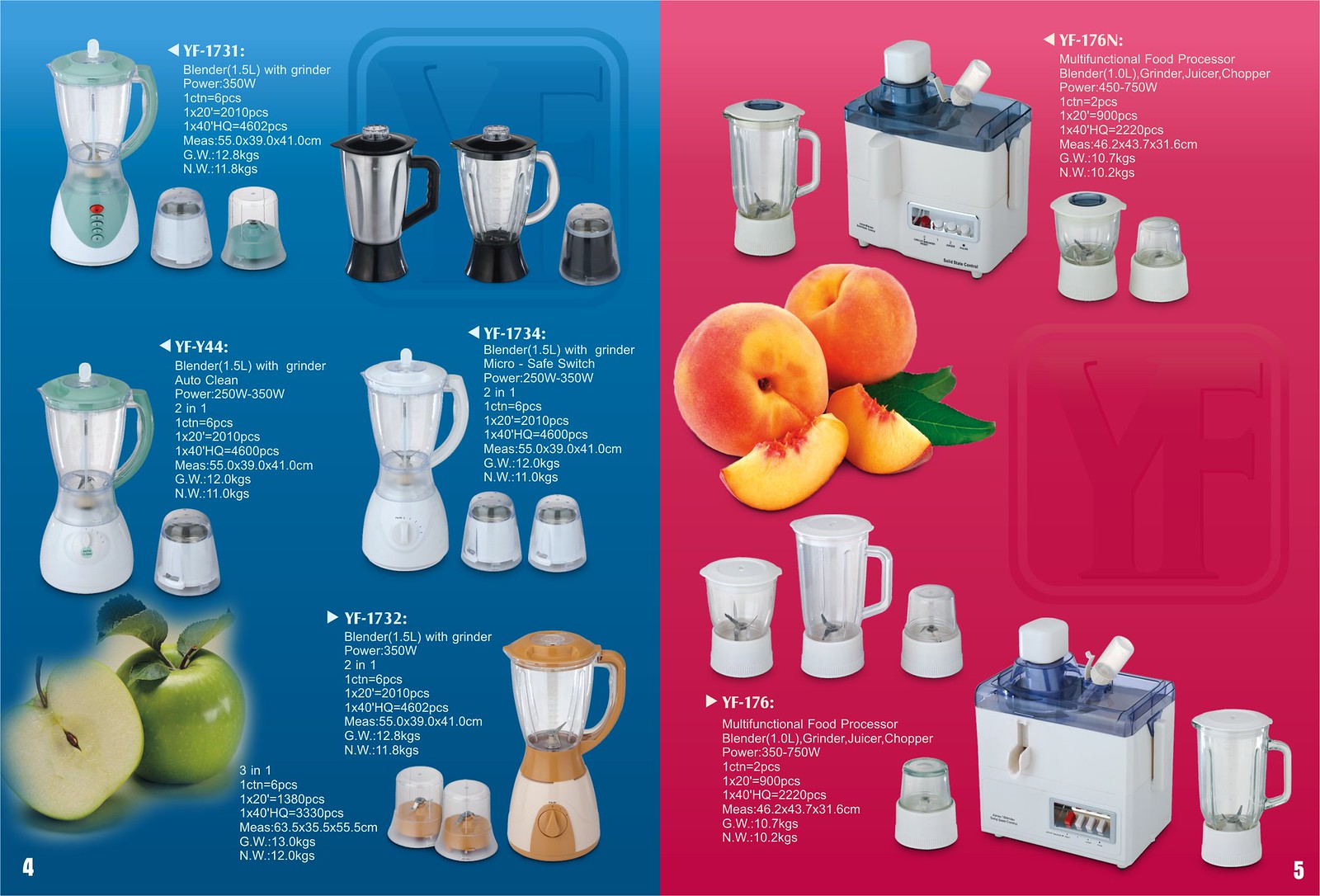This is a detailed double-page advertisement from a catalog displaying various kitchen countertop appliances against distinctly colored backgrounds. The left page has a turquoise blue background and features several white blenders, each with attachments and white print detailing their specifications. Among these are models YF1731, YFY44, YF1734, YF1732, and YF176N. In the bottom left corner, there is a photograph of a green apple and a half-sliced green apple. 

The right page, set against a pink background, showcases more kitchen appliances, including a white plastic food processor (model YF176) and its attachments, smaller food choppers, and a white toaster. The centerpiece of this page is an image of a pair of peaches and two peach slices. The spread is organized in three horizontal lines of images depicting the blenders and food processors, emphasizing the appliances' variety and functionality.